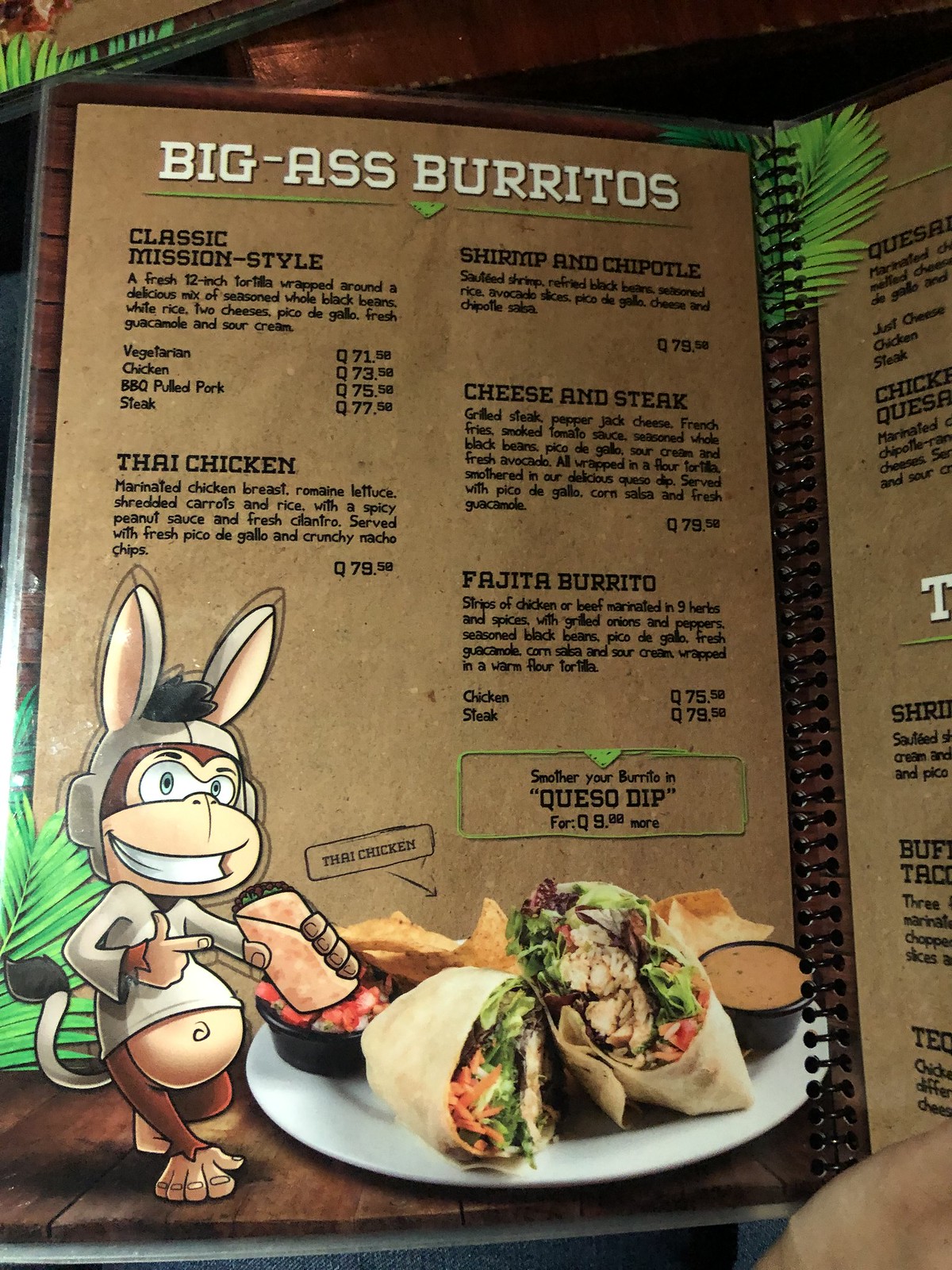The image is a photograph, taken in portrait mode, of a menu being opened inside a restaurant. In the upper left-hand corner, part of the restaurant’s wall and matching light green decorations are visible, suggesting coherence with the decor inside the menu. There appears to be another menu or some other item behind it.

In the bottom right-hand corner, a light-skinned hand is seen holding the menu open. The menu itself resembles a spiral notebook with black rings binding the plastic-protected cardboard pages. This plastic cover is intended for durability and easy cleaning.

At the top of the menu, bold text reads "Big-Ass Burritos." Below this heading, the menu is divided into two columns. The left column is titled "Classic Mission Style," describing a fresh 12-inch tortilla filled with seasoned whole black beans, white rice, two cheeses, pico de gallo, fresh guacamole, and sour cream. Various filling options are listed below: vegetarian, chicken, BBQ pulled pork, and steak, with corresponding prices in an unfamiliar currency (Q 71, 58 73, 50 75, 15 77, 50).

Underneath this section, there’s a description for "Thai Chicken," which includes marinated chicken breast, romaine lettuce, shredded carrots, rice, spicy peanut sauce, fresh cilantro, pico de gallo, and crunchy nacho chips, priced at Q79.

In the bottom left-hand corner of the image, there is a whimsical illustration of a monkey in a rabbit costume next to actual photographs of burritos on a plate, served with sauces and nacho cheese. A small rectangular section labeled "Thai Chicken" with an arrow points towards the burrito description, assisting with identification.

The second column of the menu starts with titles like "Shrimp and Chipotle," "Cheese and Steak Fajita Burrito,” each followed by their detailed descriptions and prices. There is also a prominent green rectangle offering the option to "Smother your burrito in queso dip for Q9 more."

On the upper right extending towards the lower part of the image, the edge of the second page is visible, indicating sections for "Quesadillas," "Chicken Quesadilla," and potentially a "Shrimp" option, hinting at the diversity of dishes available in the menu.